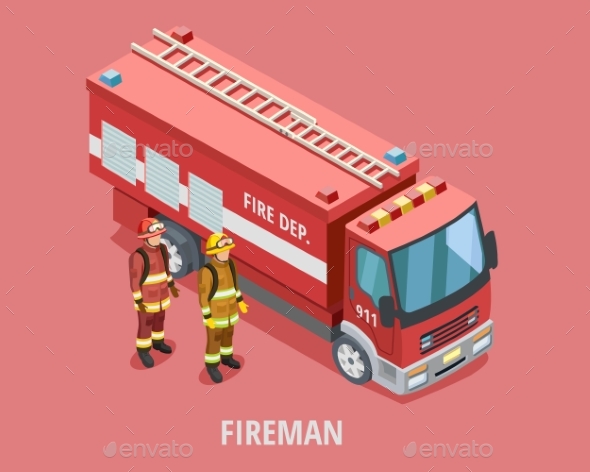The image is a cartoon-style illustration set against a solid dark pink square background, with a light gray watermark that says "Envato." Diagonally spanning from the upper left to the lower right corner of the image is a red fire truck, prominently displaying the words "FIRE DEP." and the number "911" in white on its side. The truck has a large front window, black side mirrors, and a gray bumper. Attached to its red top are two gray ladders. Two firemen stand in front of the truck, positioned in the lower left segment of the image. One is wearing a dark red uniform and hat, while the other is wearing a yellow uniform and hat. Centered at the bottom of the image, in large white capital letters, is the word "FIREMEN."